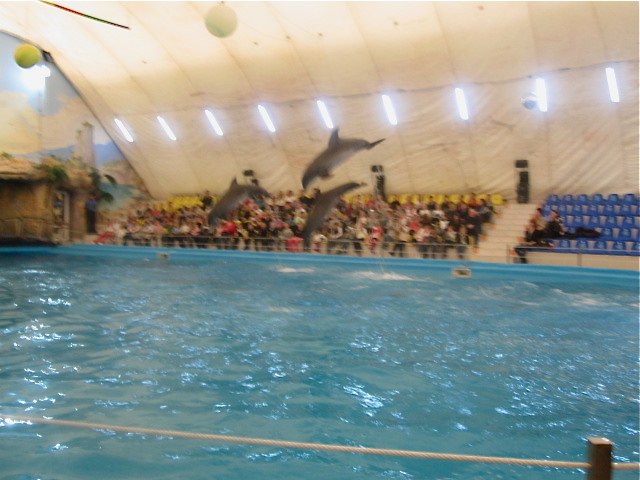This photo captures a dynamic moment at a large aquatic park, reminiscent of SeaWorld. The scene features three dolphins leaping out of a vast, bright blue pool, suspended mid-air and about to dive back in. The motion blur of the dolphins signifies their swift, synchronized jumps. The enclosure, likely made of canvas, resembles a giant tent with vertical slits, filtering light into the space. A densely packed bleacher section extends across the middle of the image, teeming with spectators, while a smaller, sparsely populated section with blue seats lies off to the right. Above the pool, the tent's interior displays a mural to the upper left and sports a few suspended balls, not directly interacting with the dolphins. Overall, the image endeavors to capture the excitement and grandiosity of the performance amidst the blue expanse of the tank, creating a vibrant, albeit slightly chaotic, snapshot of the aquatic spectacle.